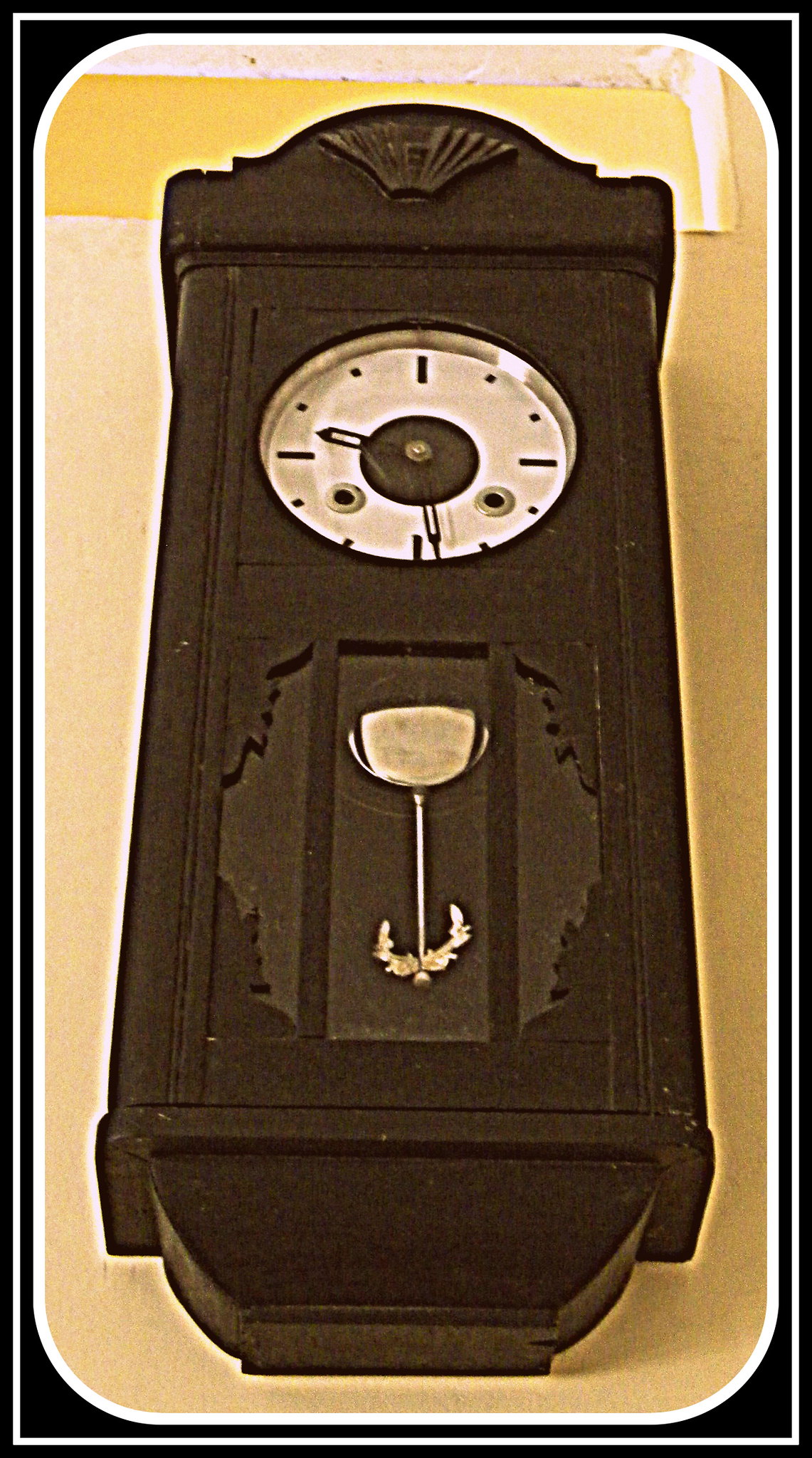"This image depicts an antique wall clock, meticulously crafted from rich, dark wood. The clock features an elongated, slender design adorned with intricate ornamental details that enhance its vintage charm. Notably, the clock face is devoid of traditional numerical markers, instead relying on elegantly designed hands, which are currently positioned at approximately 9:28. There is an intriguing metal component visible at the front of the clock, suggesting the possible presence of a pendulum, though it's unclear if it is functional. The clock is presented within a photograph that is artistically bordered with a sleek black frame accentuated by a thin white line, and the overall composition is softened by gracefully curved corners, adding a touch of modern sophistication to the image's presentation."